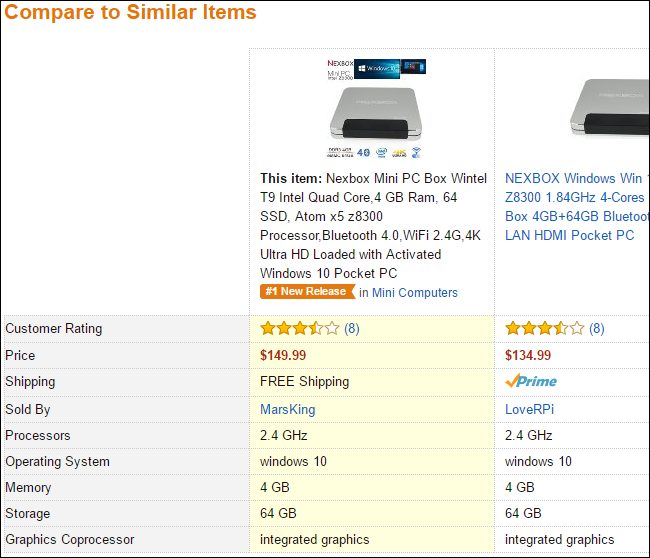Here is a cleaned up and detailed descriptive caption based on the provided voice description:

---

This image is an Amazon advertisement showcasing a user rating comparison between different products. At the top left, highlighted in orange, is the text "Compare to similar items." Below this, there is a horizontal lineup of various products available for comparison. 

The focal product is an Xbox Mini PC Box—Wintel T9. This mini PC features an Intel Quad-Core processor, 4GB RAM, and a 64GB SSD. It supports Bluetooth 4.0, Wi-Fi (2.4G), and delivers 4K Ultra HD resolution, preloaded with an activated Windows 10 operating system. This product is labeled as the 'Number One New Release' in the mini computer category.

Beside this product, there is a comparison with another item, the NextBox Windows WIN. Both products have received an eight-star customer rating. The Xbox Mini PC Box is priced at $149.99 with free shipping, and is sold by Mars King, while the NextBox Windows WIN costs $134.99, is available with Amazon Prime shipping, and is sold by Love RPI.

Following the product listings, there is a detailed comparison which includes information on their processors, operating systems, memory capacities, storage options, and graphic coprocessors.